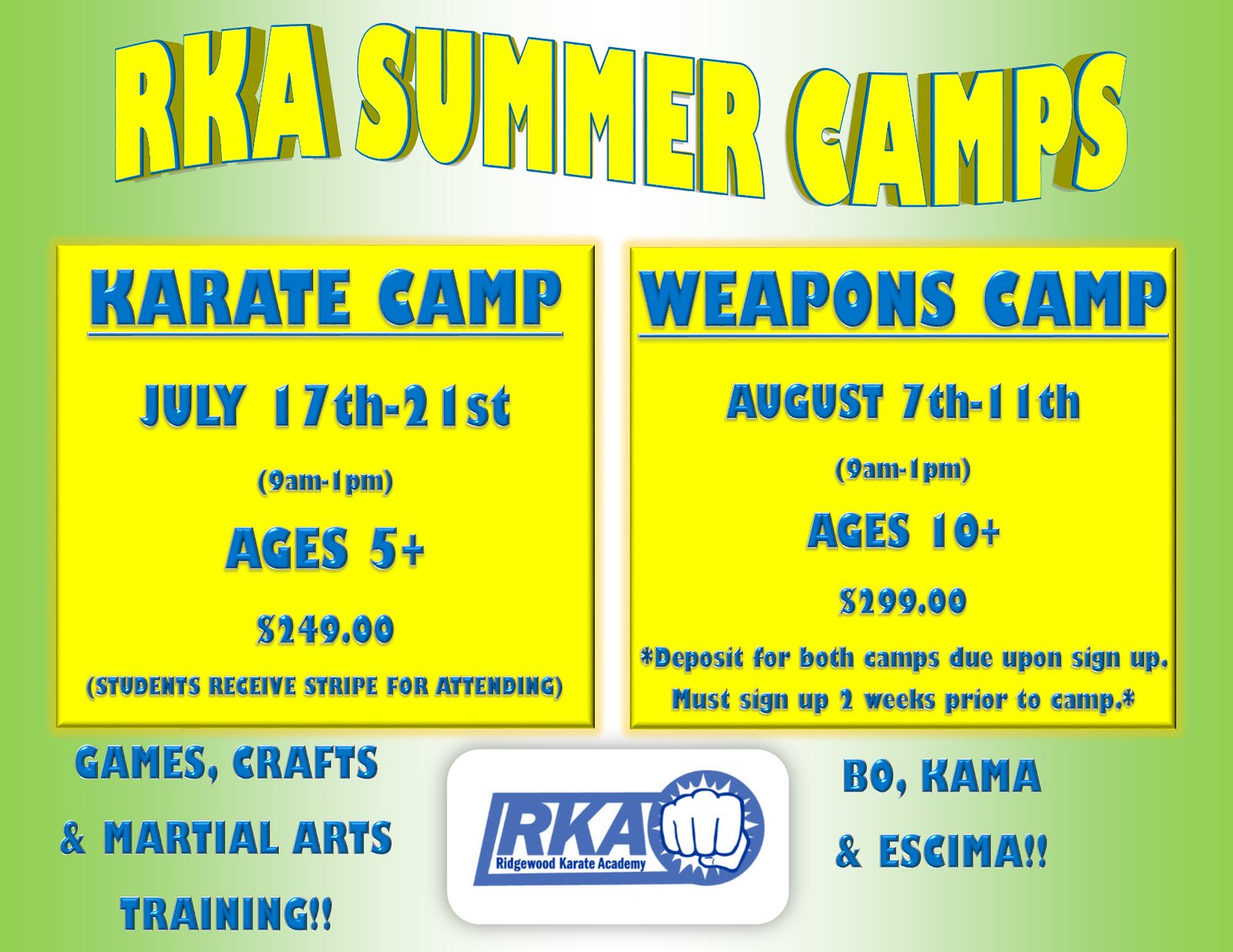This advertisement for RKA Summer Camps features a gradient green background, transitioning from light at the center to darker green on the edges. At the top, bold yellow text with a blue outline and gray shadow reads "RKA Summer Camps" in a slightly wavy pattern. Below are two yellow rectangles with blue text. The left rectangle details the "Karate Camp," running from July 17th to 21st, 9 AM to 1 PM, for ages 5 and up, priced at $249. It mentions that students receive a stripe for attending. The right rectangle highlights the "Weapons Camp," scheduled for August 7th to 11th, 9 AM to 1 PM, for ages 10 and up, costing $299. It notes that a deposit for both camps is due upon sign-up and participants must enroll two weeks prior to the camp dates. Additional text outside these rectangles reads "Games, Crafts, and Martial Arts Training" on the bottom left and "Bow, Comma, and a Schema" on the bottom right, both in blue font. A white rectangle at the bottom center features a blue-outlined white fist with the letters "RKA" below it, followed by "Ridgewood Karate Academy."